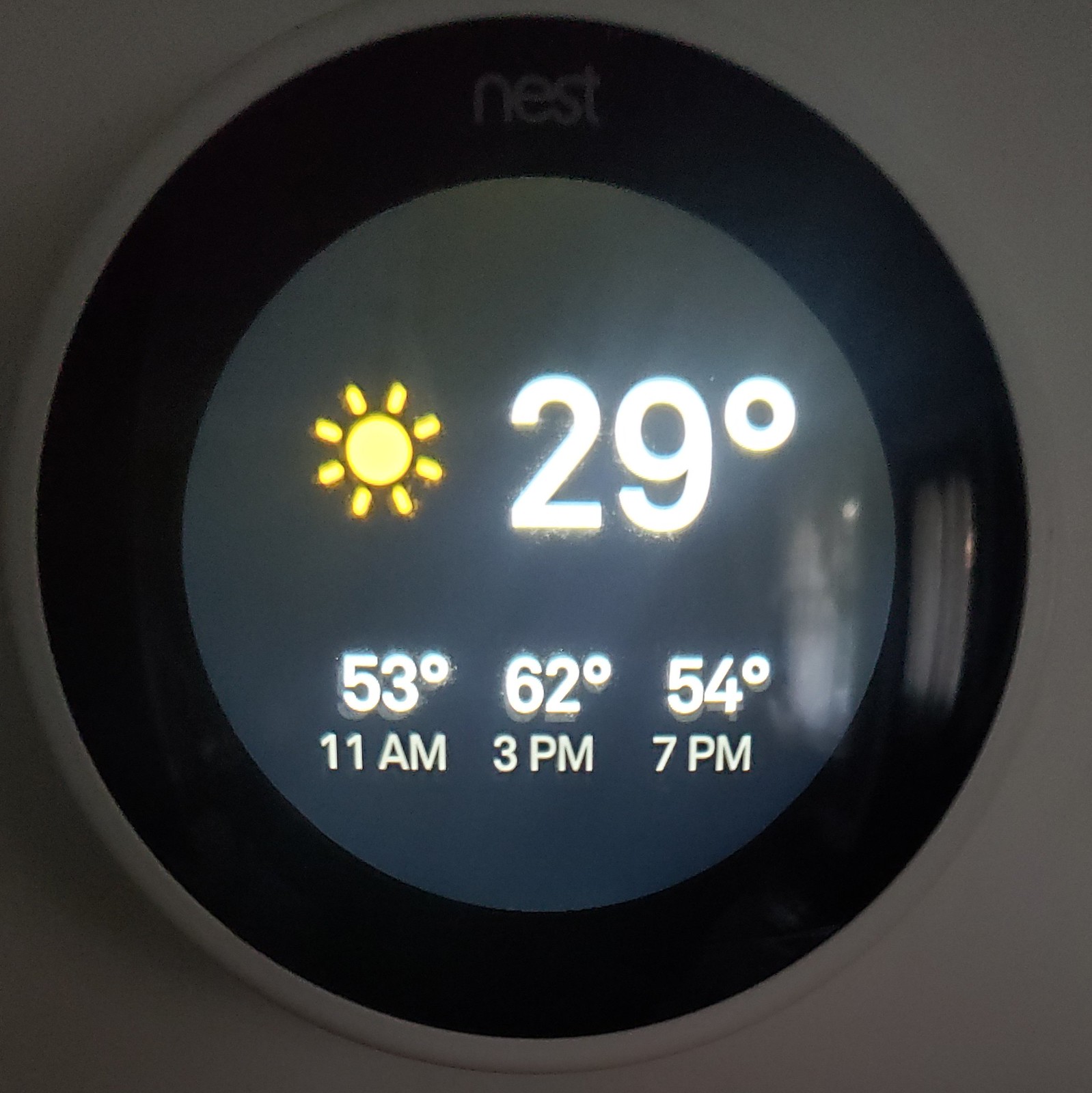A close-up image of a modern sunrise alarm clock face set against a white background. The clock features a raised white rim with a glossy black inner circle. On the right side of this black area, a reflective shine is visible. The center of the dial has a lighter gray hue, contrasting with the darker black ring. At the 12 o'clock position, faint gray lettering spells out "NEST." In the upper left portion of the dial, there's a bright yellow sun icon with rays radiating outward, symbolizing sunrise. Nearby, large white numbers display "29°", with a degree symbol positioned above and to the right of the number 9. Below this, three separate entries are listed: "53°" at "11 a.m.," "62°" at "3 p.m.," and "54°" at "7 p.m.," all in white text. The combination of detailed iconography and vibrant data creates a vivid and informative clock face.